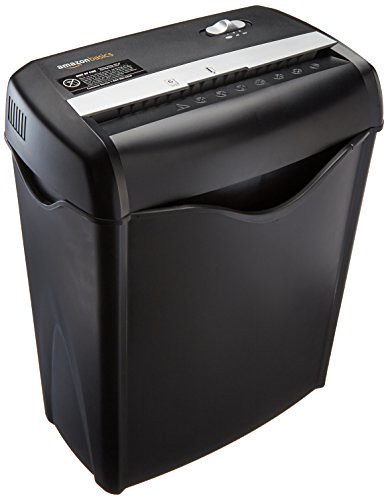This photograph showcases a black Amazon Basics paper shredder in a three-quarter view from above, prominently featuring its front, right side, and top. The shredder consists of a black wastebin at the bottom and a detachable top section. The top section houses various controls and settings, including a silver-colored bar that marks the paper inlet and a toggle button in the upper right corner that switches between "off," "on," and "reverse" modes. There is a visible warning sticker with icons indicating what should not be placed in the shredder. The brand name "Amazon Basics" is prominently displayed on the upper left of the shredder's top. The background of the photo is white, emphasizing the product's sleek design and new condition. The bottom section of the shredder features a slight opening to facilitate easy removal of the wastebin. Despite the detailed icons and warning label present, no power cord is visible in this image.